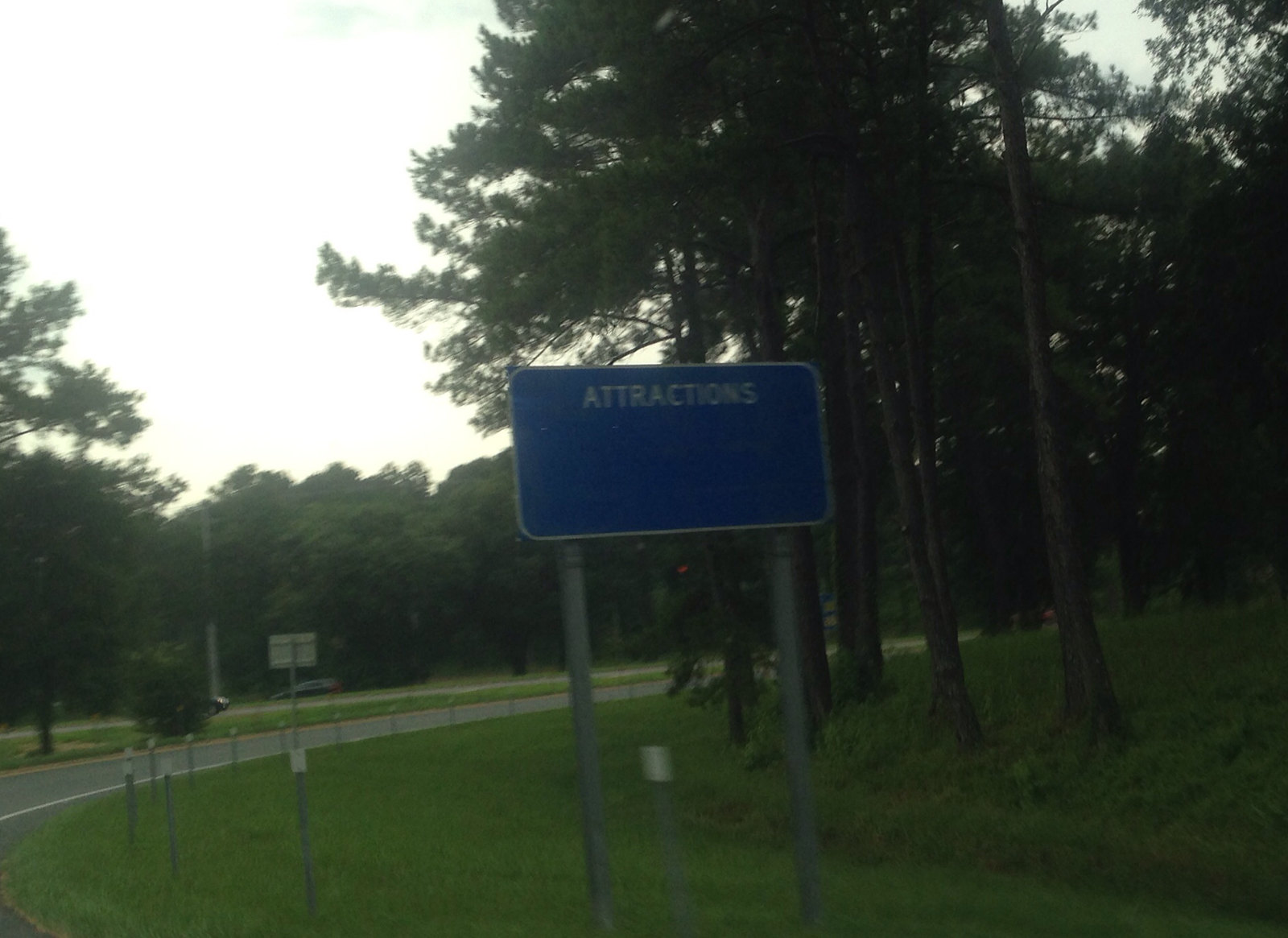The image captures a seemingly tranquil scene from what appears to be outside a car window. Dominating the lower right quadrant, there's a green field that smoothly transitions into a curving asphalt road toward the left side of the frame. Lining this road, metal signposts with white reflective tabs stand a few feet into the grassy area, suggesting the presence of a guardrail. Central to the composition is a blue rectangular sign mounted on two sturdy poles, bearing the white text "ATTRACTIONS" in capital letters. The surroundings are largely wooded, with tall trees flanking both sides of the road, reinforcing the impression of a forested area or park. The road extends from the left periphery and seems to merge into a highway or an on-ramp, hinting at a rest area nearby. The image carries a subdued, late-afternoon ambiance, with minimal sunlight filtering through, signaling the approach of dusk.